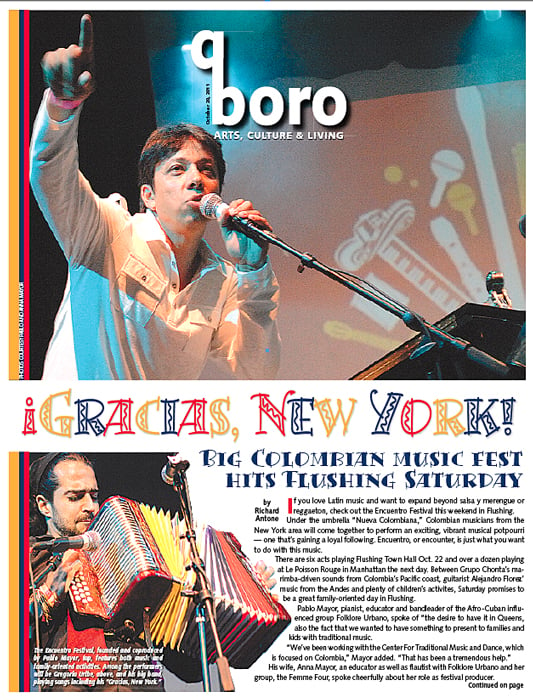In this vertically oriented, magazine-style photograph, a young man, likely in his late 20s or early 30s, dominates the scene. Seated in front of a microphone positioned near his mouth, he points upwards with his right hand, as if emphasizing a point. He has brown hair, fair skin, and wears a long-sleeved white shirt, presenting a clean and professional appearance.

The top section of the image is overlaid with text, indicating it is a cover or an advertisement. The header reads, "Q Borough, Arts, Culture, and Living," establishing the theme of the content. Just beneath this, in vibrant, varied fonts, the text announces, "Gracias, New York. Big Colombian Music Fest hits Flushing, Saturday." 

Following this, more detailed text is visible, stating, "If you love Latin music and want to expand beyond salsa and merengue, check out the En Suento Festival this weekend in Flushing under the umbrella Nueve Colombiana." The advertisement effectively showcases an upcoming cultural event, appealing to those interested in diverse Latin music experiences.